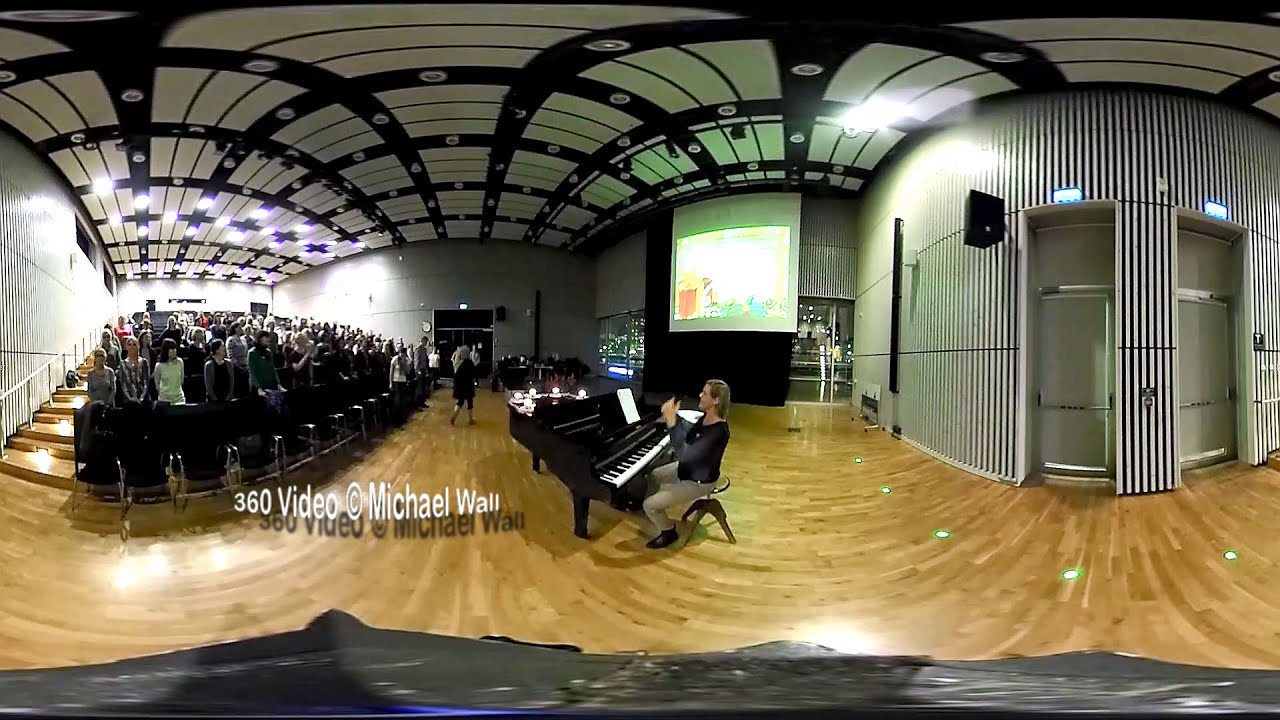The image is a panoramic view of the interior of an auditorium, taken with a technique that causes some warping and distortion. At the center of the image is a woman seated at a black grand piano, facing towards the right side of the frame with a sheet of music in front of her. She is wearing a long-sleeved black shirt and grey pants, and is seated on a stool-like seat. The floor beneath her is polished light tan wood. She appears to be interacting with an audience situated to the left side of the image, who are standing in stadium-style seats. Among the audience, one woman appears to be leaving while another person is walking within the room. Behind the pianist, there is a projector screen displaying an indistinct yellow image. The walls of the auditorium are gray with white and gray acoustic panels, and the ceiling features a distinct checkered pattern of black and white with visible lights and structural lines. On the right side of the image, there are two push doors, and on the left side, there are windows and another door. In between the pianist and the audience, white text reads, "360 video at Michael Wall."